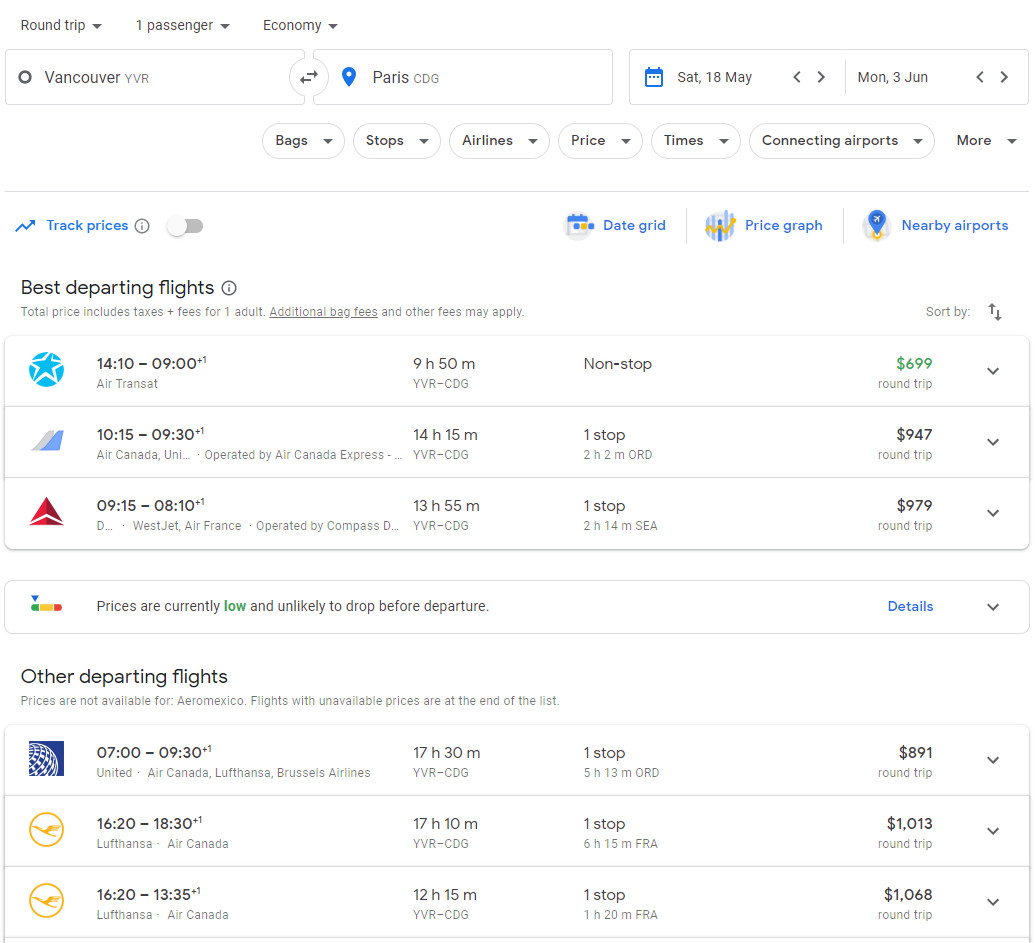The image depicts a flight search interface with a clean, white background. In the top left corner, text indicates a "Round Trip" for "One Passenger" in "Economy" class. Below this header are three horizontal search bars. The first bar displays "Vancouver," next to which is a circular icon with arrows pointing left and right. The middle search bar reads "Paris," and to its right is a blue calendar icon. The departure and return dates are shown as "Saturday, May 18th" and "Monday, June 3rd," respectively.

Below the search bars are six white tabs with black text: "Bags," "Stops," "Airlines," "Price," "Times," and "Connecting Airports," along with a "More" option that is not in a tab. Further down, on the left side, there is an option to "Track Prices," which is toggled off. Centrally, there are options displayed as "Date Grid," "Price Graph," and "Nearby Airports," each accompanied by icons.

On the left side, the section is labeled "Best Departing Flights" in black text, with smaller subtext underneath. On the right side is a "Sort By" option with an up and down arrow. Below the "Sort By" option, the "Price per Trip" is listed. Each flight entry on the left features an airline icon, departure time, and the airline name below it. To the right, the flight duration is displayed, followed by information on whether the flight is nonstop or with stops. This section contains three such listings.

A space separates this from another tab that states "Prices are currently low and unlikely to drop before departure." Below this notice, another section of departing flights follows the same layout and contains three listings.